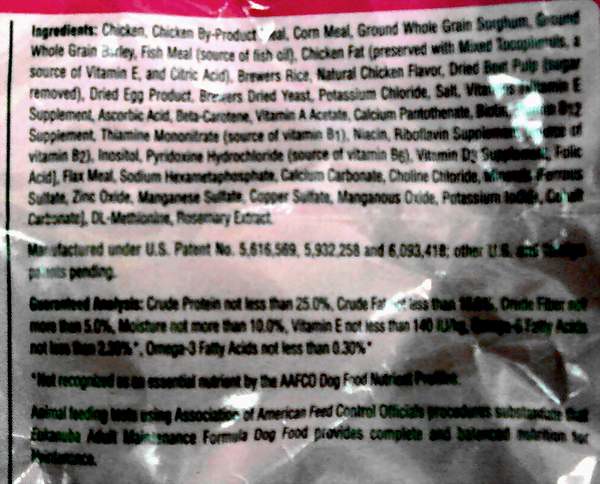The image showcases the back of a crinkled, slightly blurry plastic product label. The label features a red strip at the very top, with the remainder of the label being predominantly white. Down the left-hand side runs a thin black horizontal line. 

The top section of the label lists the ingredients, led by "chicken byproducts." Other ingredients include cornmeal, ground whole grains, sorghum, fish meal, chicken fat, natural chicken flavor, brewers rice, dried beet pulp, dried egg product, brewers dried yeast, potassium chloride, and calcium pantothenate. The list continues with numerous preservatives towards the bottom. Additionally, there is a note indicating that the animal feeding guidelines have been approved by the Association of American Feed Control Officials (AAFCO).